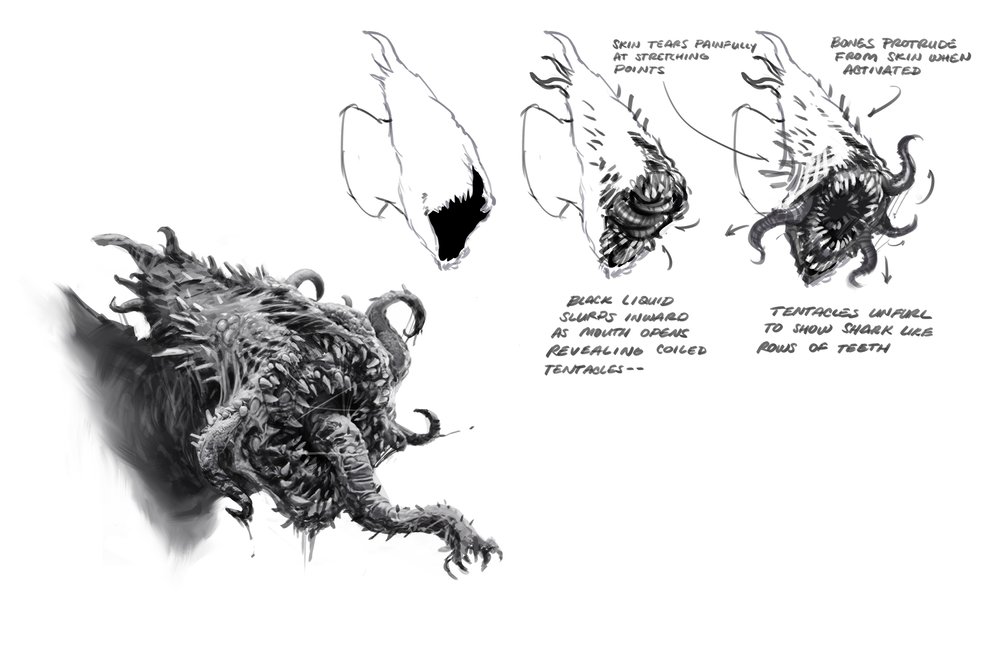The image is a detailed black and white drawing of an imagined sea creature with centipede-like characteristics. The creature has a grotesque head, coated with a myriad of fangs and teeth, and a thick neck extending into visible shoulders. Protruding from its mouth is a worm-like appendage lined with additional teeth and tentacles. At the back of its head, there is a tail-like extension and sharp curls acting as arms. 

Displayed along the top of the image are three progressive sketches illustrating the development of this creature, accompanied by descriptive text. The first sketch shows a basic outline with a mouth or an intestinal opening. The second adds more detail, including intestines and nascent tentacles. The third sketch elaborates further with fully formed feelers or tentacles, highlighting features such as sharp rows of shark-like teeth and skin that tears when stretched. The detailed descriptions note that black liquid slurps inward as the mouth opens, revealing coiled tentacles, and that bongs protrude from the skin when activated.

In the bottom left corner, beneath these three sketches, is a more detailed and finished drawing of the sea-creature, showcasing its many grotesque and monstrous features in full form, including the flesh-tearing skin, sharp curls, and the clawed hand-feeler extending from the front. The entire composition provides a thorough and gruesome depiction of this fantastical creature.